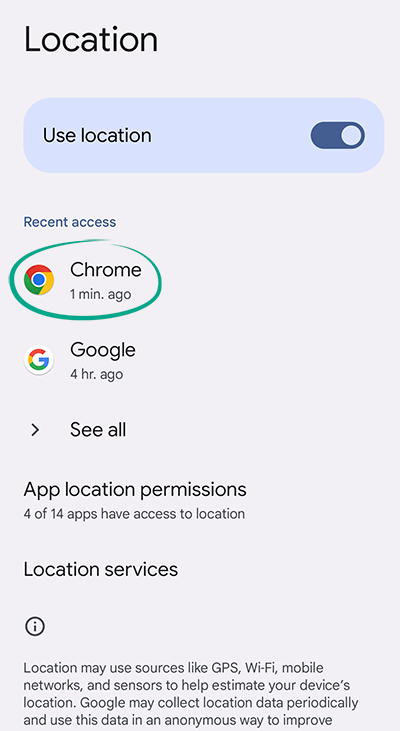This image is a portrait-mode screenshot with a solid gray background. In the upper left-hand corner, the word "Location" is displayed in bold black text. Below it, there is a section with a light blue background and rounded corners, containing the text "Use location" alongside a toggle button, which is turned on and has become dark blue to indicate its active status.

The next section, labeled "Recent Access," lists the apps that have recently accessed the device's location. This section shows that "Chrome" accessed the location one minute ago, highlighted by a green circle drawn by the screenshot's creator, and "Google" accessed it four hours ago. To the right of this, an arrow labeled "See all" indicates the option to view more details.

Further down, the section titled "App location permissions" states that "4 of 14 apps have access to location." Following this is the "Location services" section, featuring a small information icon within a circle. Below this icon is a description explaining that location services may use sources like GPS, Wi-Fi, mobile networks, and sensors to estimate the device's location, and that Google may periodically collect this data and use it anonymously to improve its services.

Given the information and the green circle around the "Chrome" entry, it appears that the person who took the screenshot might be concerned or surprised that Chrome accessed their location one minute ago, while the "Google" entry from four hours ago was not highlighted, suggesting they are either less concerned about or aware of Google's periodic location access.